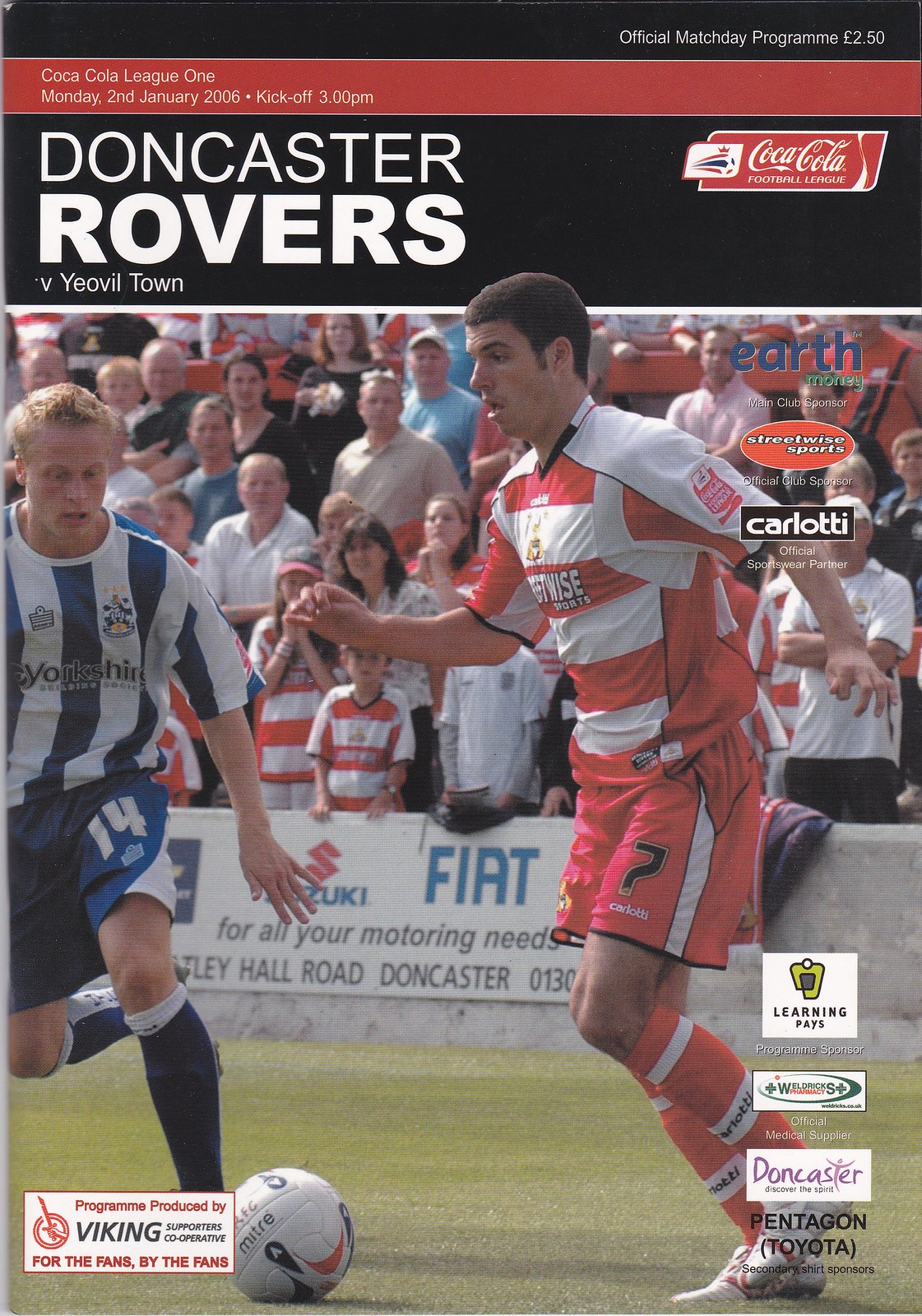The cover of this full-color magazine is dedicated to a soccer game featuring the Doncaster Rovers. Across the top, there’s a sleek black banner with a thin red line running horizontally. Above this red line, white text reads “Official Match Day Program L2.50” (or 2.5 Euro). The red banner itself states “Coca-Cola League 1” in white print, accompanied by the date “Monday, January 2, 2006,” and “kickoff 3 p.m.”

Dominating the center, “Doncaster Rovers” is displayed prominently in large white text against the black background, followed by “v. Yeovil Town.” To the right of this text is a Coca-Cola Football League logo. Beneath these headings, the main image captures the energy of the match, depicting two players in action against each other: one in a blue and white uniform and the other in red and white. The soccer ball they contend for, primarily white with red and blue accents, is visible near the bottom of the image. The backdrop features bleachers filled with spectators.

Additionally, the cover includes various sponsor logos, predominantly arranged along the right side of the cover with at least one on the lower left side, adding to the commercial look and feel of the program.